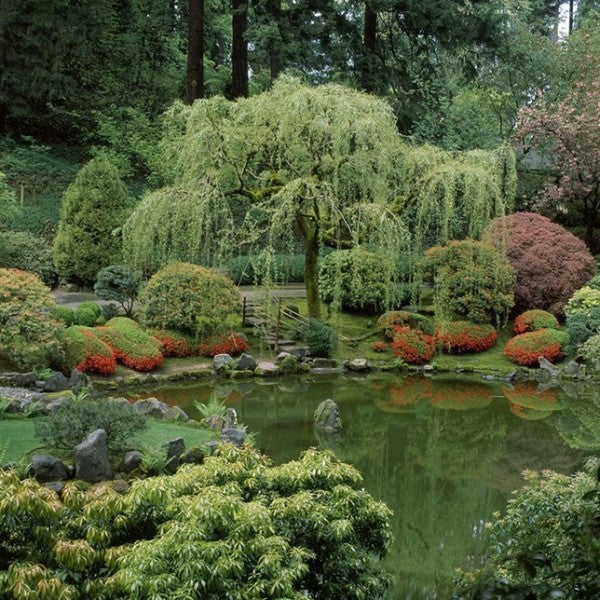The image showcases a meticulously managed garden area with a serene, natural ambiance. Dominating the scene is a weeping willow tree with cascading branches, situated centrally by a tranquil pool with green water. This pool, bordered by an array of large stones, beautifully reflects the surrounding greenery and vibrant shrubbery. Pink bushes and additional trees enhance the garden's lushness, while concrete steps with a black railing lead up to a pathway, guiding the eye through the picturesque landscape. The background features more towering trees and a window peeking from a nearby building, hinting at an adjoining street. The overall scene, filled with bright, full flowers, exudes an air of careful cultivation and tranquility.